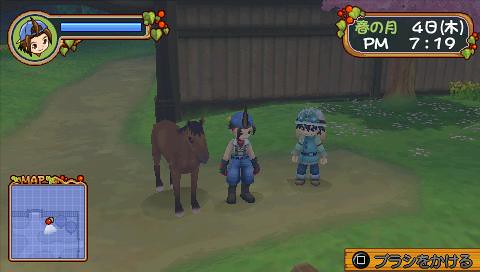This screenshot from a video game captures a vivid and dynamic scene brimming with detail. Dominating the image are two cartoonish humanoid characters standing side by side on a light tan pathway bordered by lush green grass. Both characters, with light skin and medium-length dark brown or black hair, are dressed identically in blue pants. Strikingly, they stand as tall as a nearby dark brown horse, which sports a black mane and black legs. 

The backdrop features a rustic brown wooden building, adding to the scene's quaint charm. At the top right and bottom right corners, text in what appears to be Japanese or Chinese lends an authentic touch of East Asian culture. The top left corner showcases a close-up of one character's face beside a blue experience or health bar, indicating vital statistics. Meanwhile, the bottom left corner is occupied by a detailed blue and white grid-patterned map, aiding navigation. A time indicator is subtly positioned at the top right, completing the immersive and meticulously crafted in-game environment.